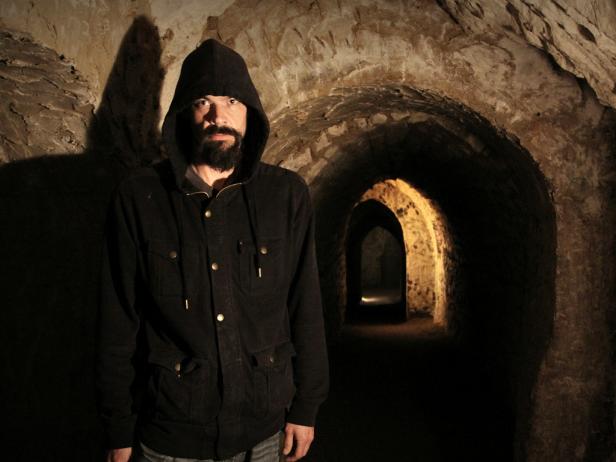In the image, a Caucasian man with a scraggly black beard and mustache stands in a dark, arched hallway, possibly underground, resembling the catacombs of Europe. He wears a close-fitting black jacket with the hood partially pulled over his head, a dark green t-shirt, and denim blue jeans. Positioned towards the left of the wide, vertical, rectangular image, the man is seen from the waist up with his arms down at his sides. Behind him, the dark cave-like tunnel, made of brown rock or clay, stretches into the distance with multiple rounded, arch-shaped doorways. A subtle gold light illuminates the back of the tunnel, enhancing the mysterious atmosphere by casting large shadows on the narrow hallway.